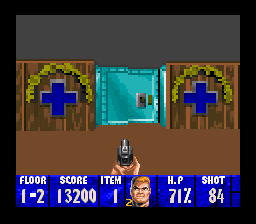Screenshot from a first-person shooter video game, featuring a central light blue vault door, flanked by wooden paneling with royal blue crosses and laurel decorations. In the foreground, a player's hands are visible, gripping a gun. Below is the score interface, displaying: Item 1, Score 13200, Floor 1-2, HP at 71%, and shots fired (84).